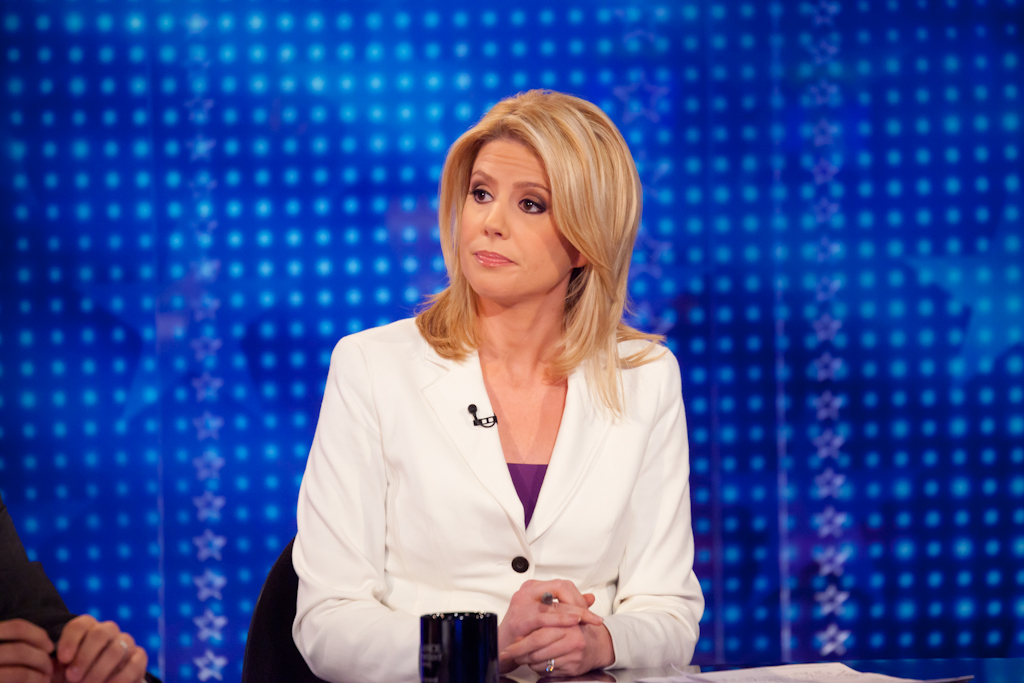The image captures a female news reporter seated at a news desk. She is dressed in a white jacket with a lower-cut purple shirt underneath. A dark microphone is pinned to her jacket lapel, and a dark button fastens her jacket. Her golden hair frames her face as she looks to her right. She has her hands folded on a reflective table, in front of which sits a black coffee mug adorned with white text. Accompanying the mug are white papers scattered nearby. She's seated on a black chair, and there's a partial view of another person's hands and body to her left. The backdrop behind her is a darker blue with organized rows of white dots interspersed with some flower shapes.